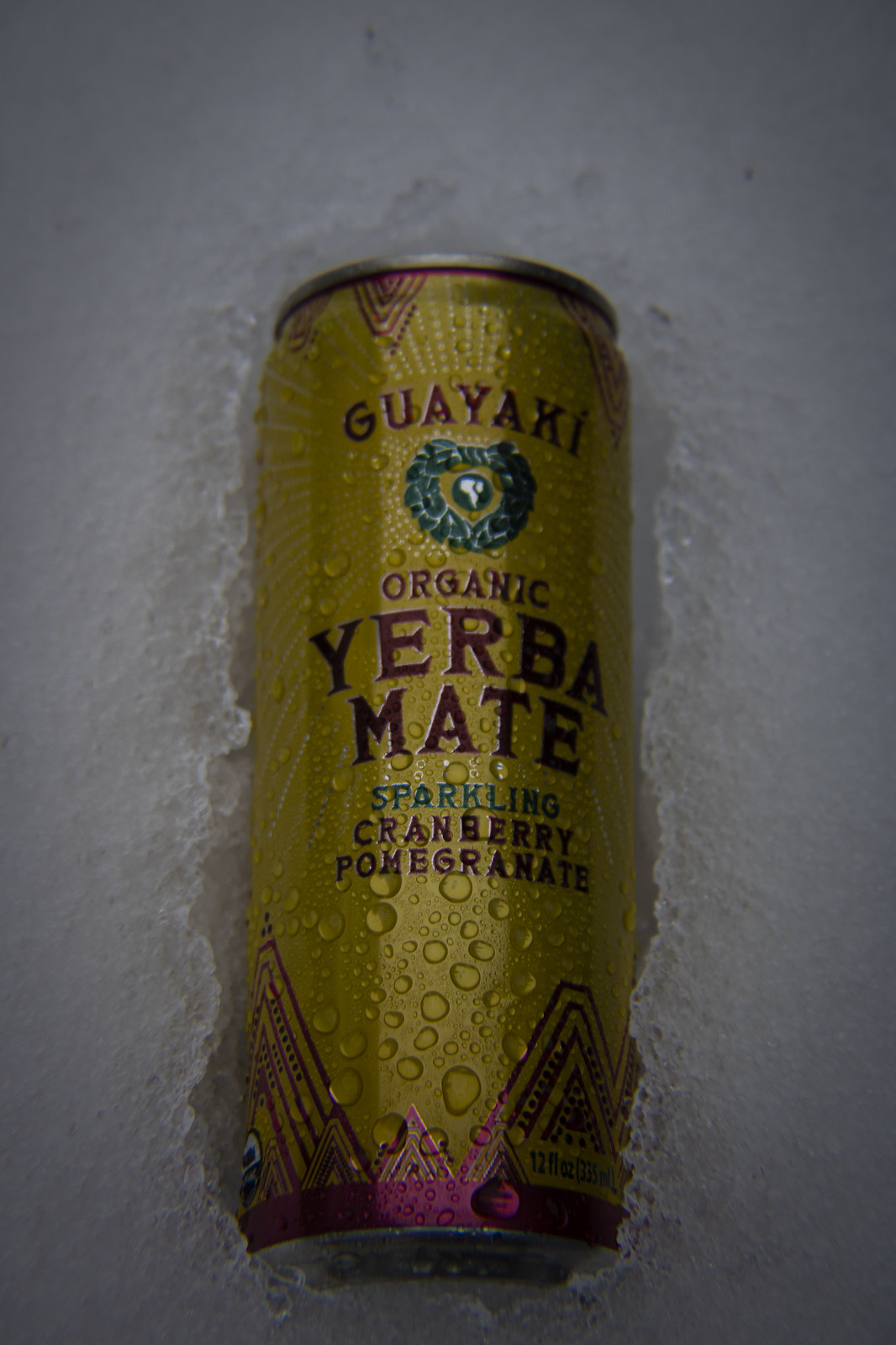The photograph captures a gold cylindrical beverage can, branded with the red text "GUAYAKI" across the top. The can, which sits amidst a surrounding of solid, well-defined icy water, is adorned with a central green wreath logo resembling the shape of Africa. Below the logo, the text reads "Organic Yerba Mate," followed by smaller green text that says "Sparkling," and finally "Cranberry Pomegranate" in black. The can is highlighted with silver-edged black font and features droplets of moisture on its surface, accentuating its cold appearance. It rests in a pool of dimly lit crushed ice, creating a distinctly chilly and refreshing visual.